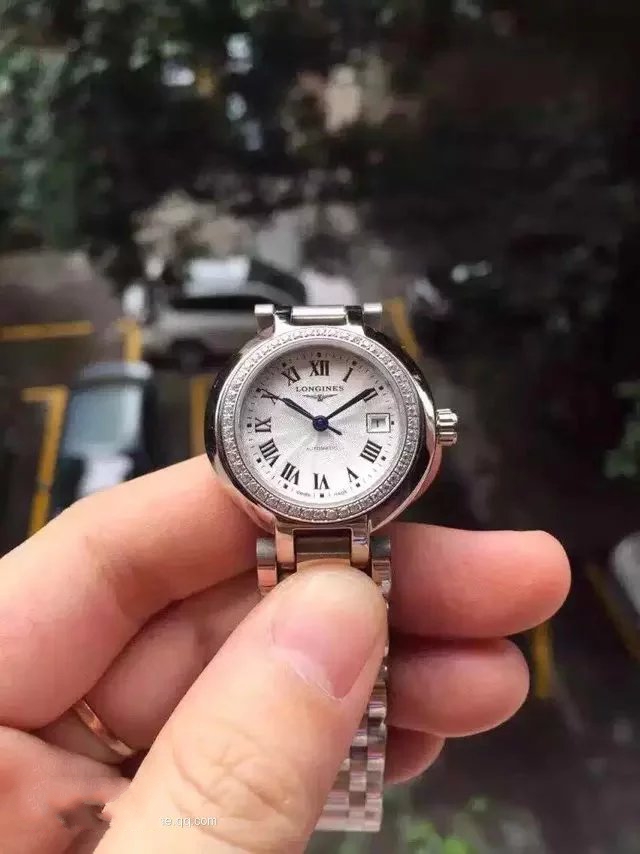In this image, a medium to light-skinned left hand holds a silver-toned watch. The thumb and the tips of the first two fingers are visible, partially wrapped around the watch and band. The person wears a gold band ring on their ring finger. The watch, which appears to be a woman's style due to its small size, features a circular, analog design with a silver metal band and Pave set diamonds around the bezel. The white watch face displays black Roman numerals, though the numeral three is replaced by a small square showing the date, and the brand "Longines" is written beneath the 12 o'clock mark. The watch's black hour and minute hands point to 10:10, and there is no second hand. The background of the image is blurred, revealing vague details of green trees and possibly a brown fence or parking lot with yellow dividing lines and a couple of cars.